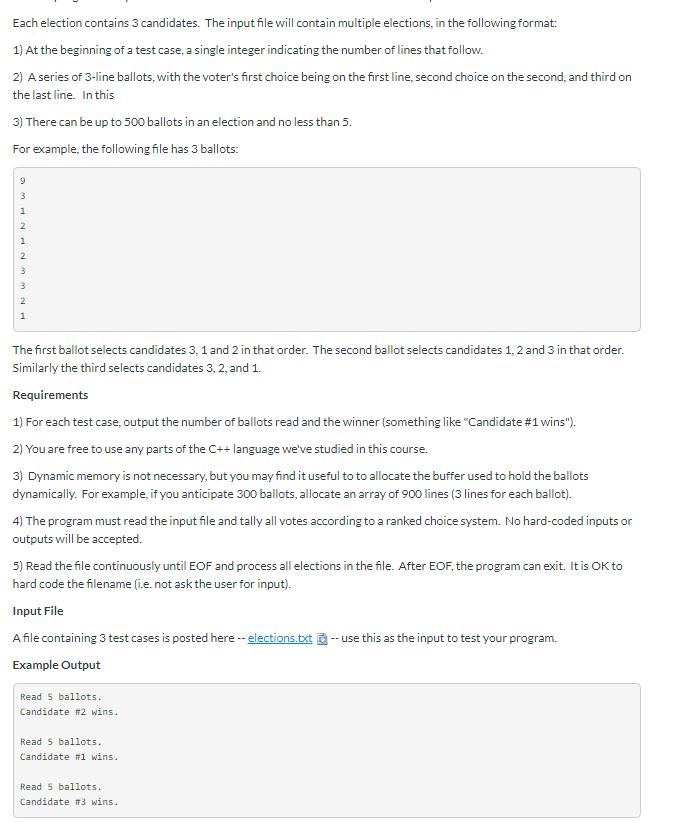The image displays a webpage that serves as an instructional guide for processing election ballots using the C++ programming language. The webpage has a minimalistic black-and-white theme with black text on a white background. The textual content details the format and structure of multiple elections, each containing three candidates.

The document starts by outlining the input file's format for the test cases:
1. At the start of each test case, a single integer indicates the number of lines that follow.
2. A sequence of three-line ballots follows, where each line represents the voter's first, second, and third choices, respectively.

The webpage specifies that each election can have up to 500 ballots but no fewer than five. For example, it includes a sample file containing three ballots, demonstrating the format:
- The first ballot selects candidates in this order: 3, 1, 2.
- The second ballot selects candidates in this order: 1, 2, 3.
- The third ballot selects candidates in this order: 2, 3, 1.

An accompanying gray box shows line numbers along the left-hand side, helping illustrate the format visually. The instructions continue to explain that for each test case, the program should output the number of ballots read and announce the winning candidate, such as "Candidate number 1 wins."

The webpage emphasizes the allowance of any C++ language features studied in the course. While dynamic memory allocation is not required, it suggests it could be useful for managing the ballots' data. For instance, anticipating 300 ballots might necessitate an array of 900 lines, with three lines for each ballot.

Overall, the page comprehensively explains how to read, process, and determine the outcomes of ballots in an election format using C++.